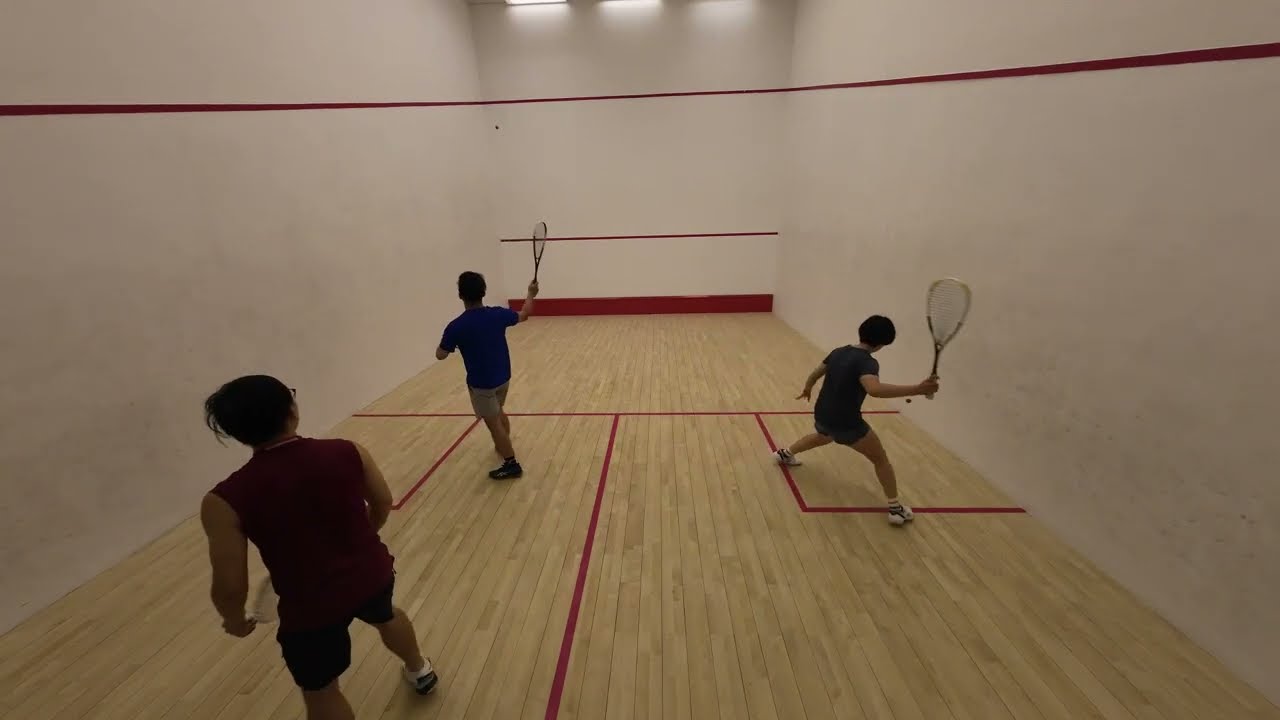In this slightly high-angle image taken from a camera mounted on a wall, we see three individuals inside a racquetball court with polished wooden floors and white walls adorned with various red lines indicating specific areas. The court features a large red line about three feet from the ceiling and another red line specific to the far wall, along with a red trim. The scene is lively with three people engaged in a game of racquetball. 

The man at the back of the court, possibly the father, is clad in a blue shirt and gray or green shorts, seemingly placing him in an instructor's role. In front of him, likely his two sons, are actively playing, with the older boy to the left wearing a dark blue shirt and black shorts and appearing around 12 to 13 years old. The younger boy, aged approximately 9 or 10, is on the right wearing a dark red shirt and black shorts, focusing on the ball that’s visible as a black dot on the court. Both boys hold racquets, poised to hit the ball in a moment of dynamic play. The younger boy is seen squatting in anticipation, while the older boy seems readying for a strike. The composition and attire dynamics, along with the likely age difference, suggest an engaging family activity.